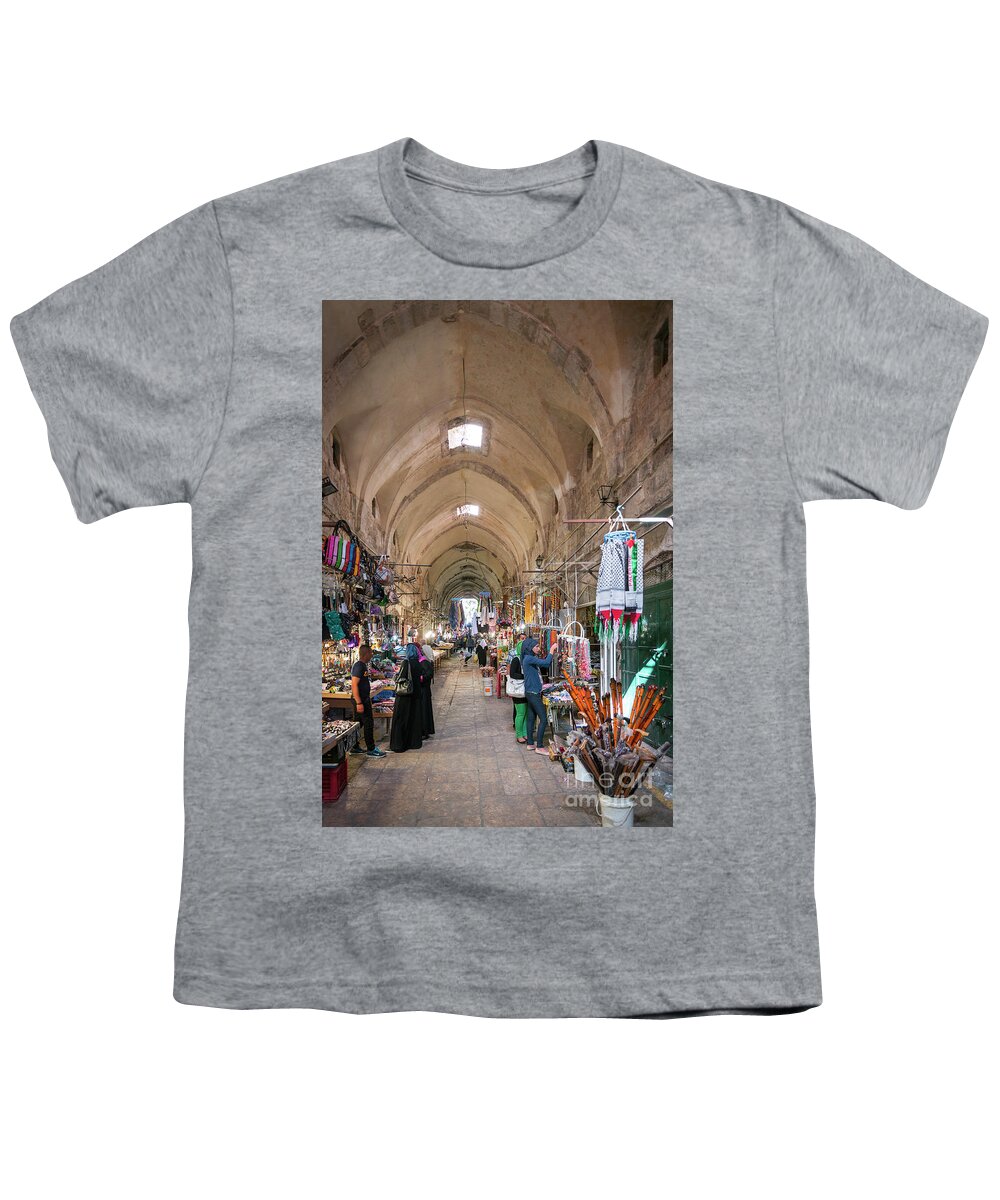The image is a detailed photograph of a plain gray, short-sleeved t-shirt on a transparent, white background. The t-shirt appears to be of lower quality and tagless. Digitally added to the shirt is a rectangle-shaped screen print featuring an intricate scene of an indoor market or alleyway with a domed, stone archway ceiling. The archway stretches towards a bright light at the end, creating a tunnel-like effect. Along both sides of the paved stone walkway, various vendors display merchandise, such as knickknacks, clothing, and bags. Sunlight filters through rectangular openings in the ceiling, illuminating the scene below. People are seen mingling along the walkway and near the stands. A watermark at the bottom right corner of the screen print reads "Fine Art America," subtly indicating the source of the image. The vibrant market depiction contrasts with the simplicity of the gray t-shirt, enhancing its visual appeal.